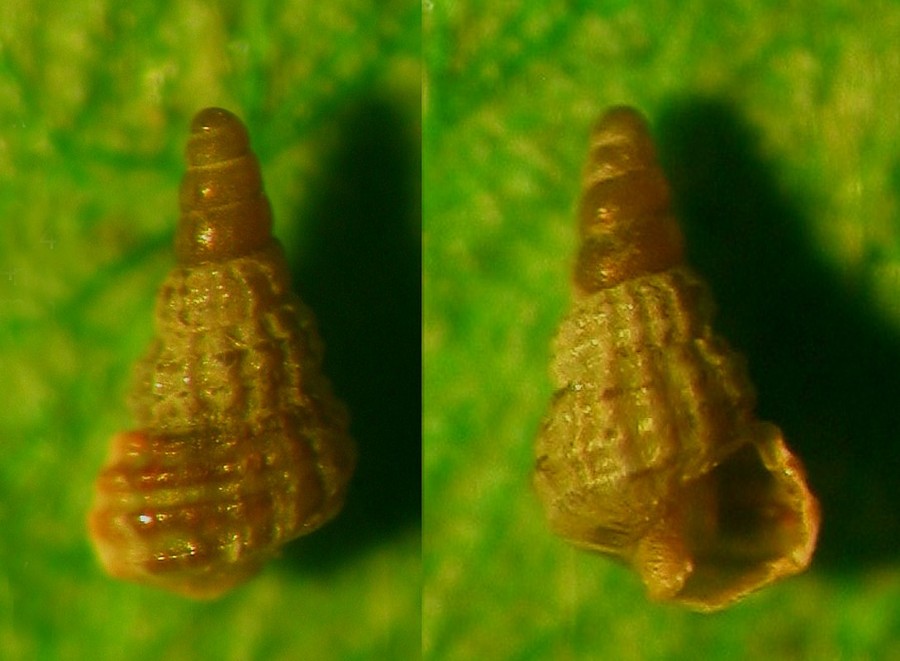This image features a small conch shell presented in a side-by-side collage on a blurred, neon green and yellow background, possibly a beach towel or a placemat. In the left image, the shell is oriented to show its amber-colored tip and textured, striated surface, which extends slightly to the left. The right image showcases the same shell flipped to display its opening, emphasizing the intricate textures visible on both sides of the shell. The imperfect lighting in the photograph casts the shell in hues of yellowish to golden brown, highlighting the darker tips and striations.